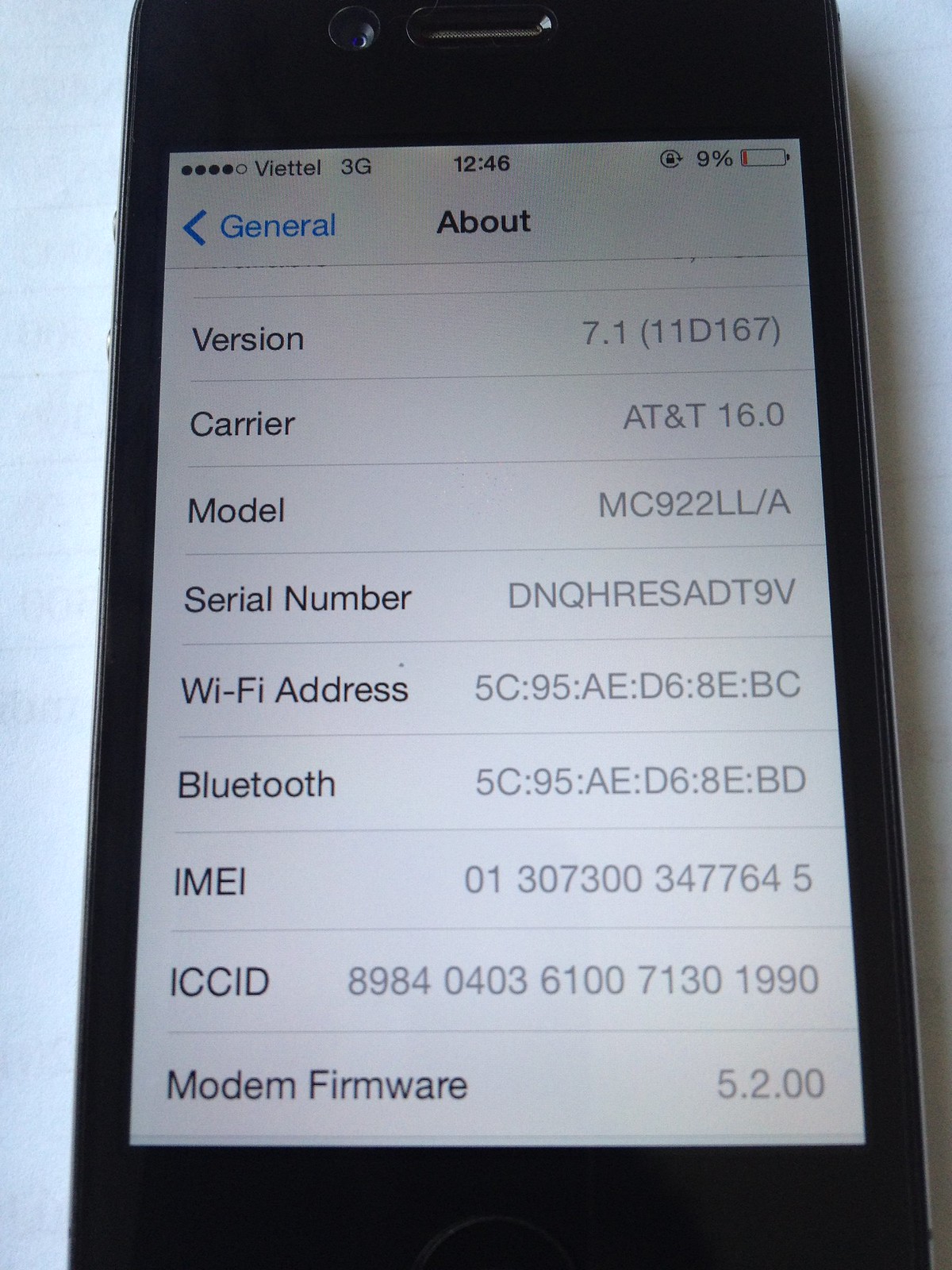The image depicts an older model iPhone with a black bezel, displaying the "About" section of its settings, indicating it is on the Viatel 3G network with 4 out of 5 signal bars. The phone shows a battery level at 9% and the time is 12:46. The top bar includes indicators for 3G connectivity and an active orientation lock. Detailed information visible on the screen includes the software version 7.1 (11D167), carrier AT&T 16.0, model MC922LL-A, and serial number DNQHRESADT9V. The Wi-Fi address is 5C:95:AE:D6:AE:BC, and the Bluetooth address shares this format but ends in BD instead. Additionally, the IMEI is 013073003477645, ICC ID is 898404038610071301990, and the modem firmware is 5.2.00. The image appears to be shot indoors, and there is a yellow "General" back button in the top left corner of the screen.